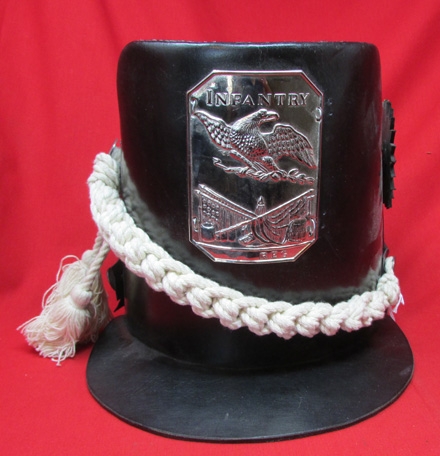The image depicts a black military hat, possibly from the U.S. War of 1812, presented against a rich red background reminiscent of a curtain or wall. The hat has a cylindrical shape, with a prominent black brim designed to shade the face. Around the base of the hat, a thick white rope is meticulously wrapped, draping elegantly to the side where it forms a knot and hangs down with two white tassels. At the center of the hat, a metallic silver insignia adorned with an eagle catches the eye. Above the eagle, the word "Infantry" is clearly engraved. Below the eagle, there appear to be two crossed swords, adding to the ornate detail. Additionally, on the right side of the hat, there is a black area that might depict a starburst design, although the details are obscured due to its position. Overall, the hat's historical significance is underscored by its elaborate design against the vivid red backdrop.